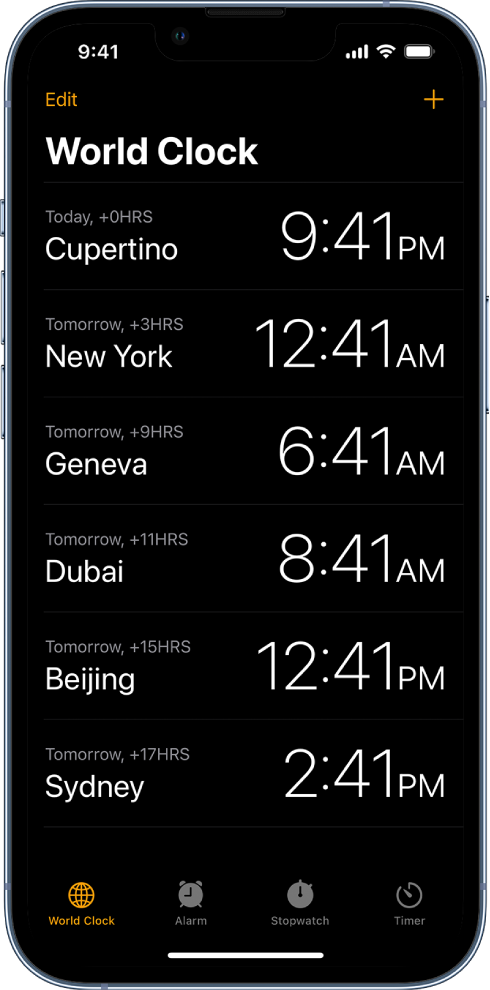The image depicts a realistic mobile phone mock-up, showcasing an app's interface set against a white background. The phone is presented front-facing, allowing a complete view from top to bottom and left to right. The device features curved corners, which adds to its modern aesthetic. 

On the screen, the background is solid black, contrasting sharply with the primarily white text and icons. The time is displayed prominently at the top center, reading "9:41". To the top-right corner, there are icons indicating full signal strength, active Wi-Fi connection, and a fully charged battery.

Below the status bar, an edit button in light orange is visible on the left-hand side, followed by a large empty space and a plus sign on the right-hand side. 

The main content area of the screen is dominated by a section labeled "World Clock" in large white letters. Underneath, the display is divided into two columns. The left column provides information about the day, time difference, and corresponding city. For instance, the first entry reads "today, +0 hours, Cupertino." 

The right column lists the local times for each respective city, with the first entry showing "9:41 PM." The subsequent rows follow the same format, detailing various cities, their time differences, and local times.

Overall, the mock-up effectively demonstrates the app's world clock feature in a clear and organized manner.